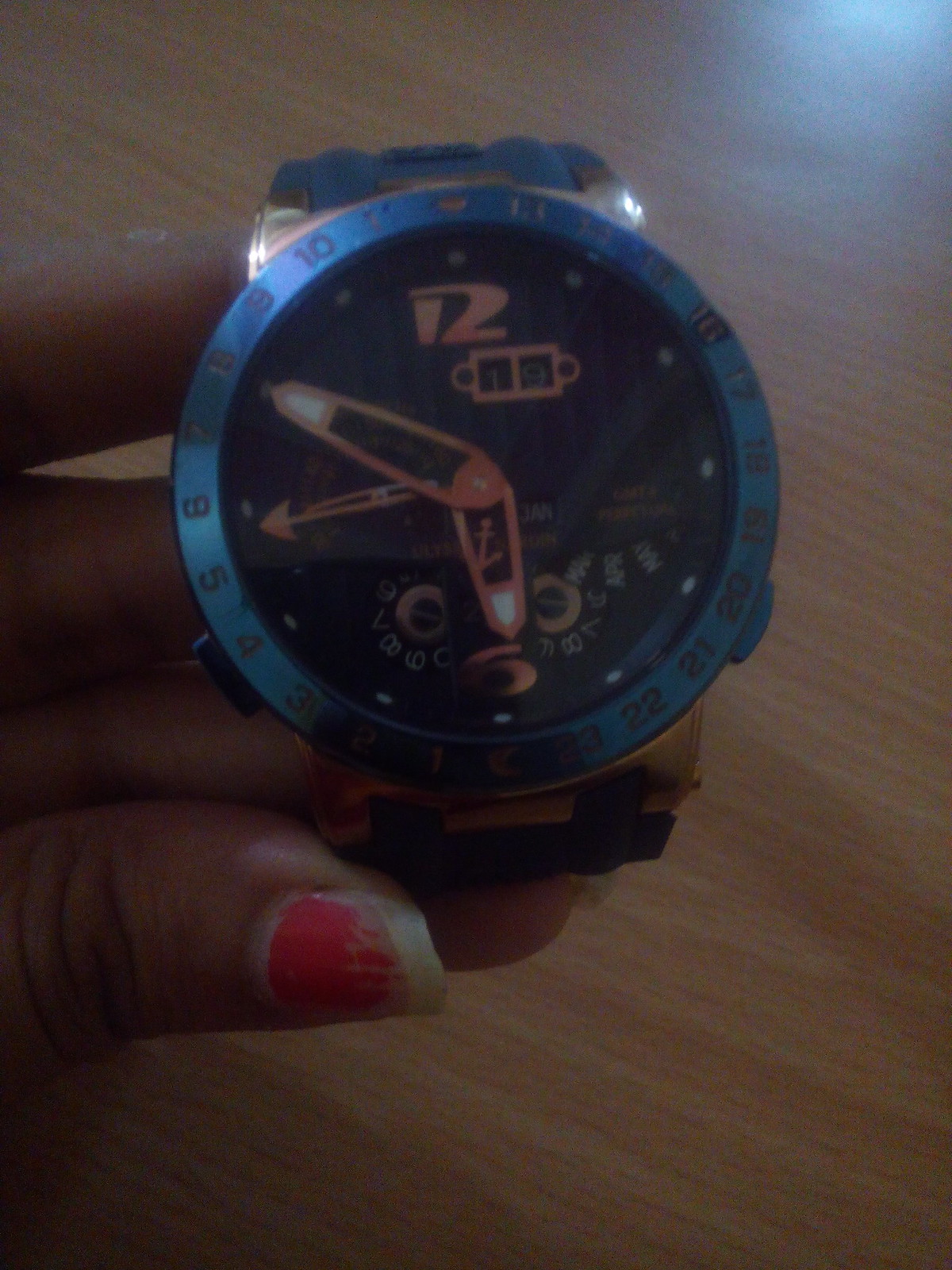In a dimly lit photograph, a close-up captures a woman's hand holding a wristwatch. Her thumb and the backs of her fingers, with a partially chipped red manicure on her thumbnail, are visible. Her dark skin contrasts the light wood laminate table on which her hand rests. The watch boasts a navy blue face encased in a striking, metallic blue frame. Its hour and minute hands are bronze, tipped with small, glow-in-the-dark segments, while the second hand is also bronze. Bold bronze numerals mark the 12 and 6 positions, and glow-in-the-dark dots indicate the rest of the hours, enhancing the watch's elegant design.